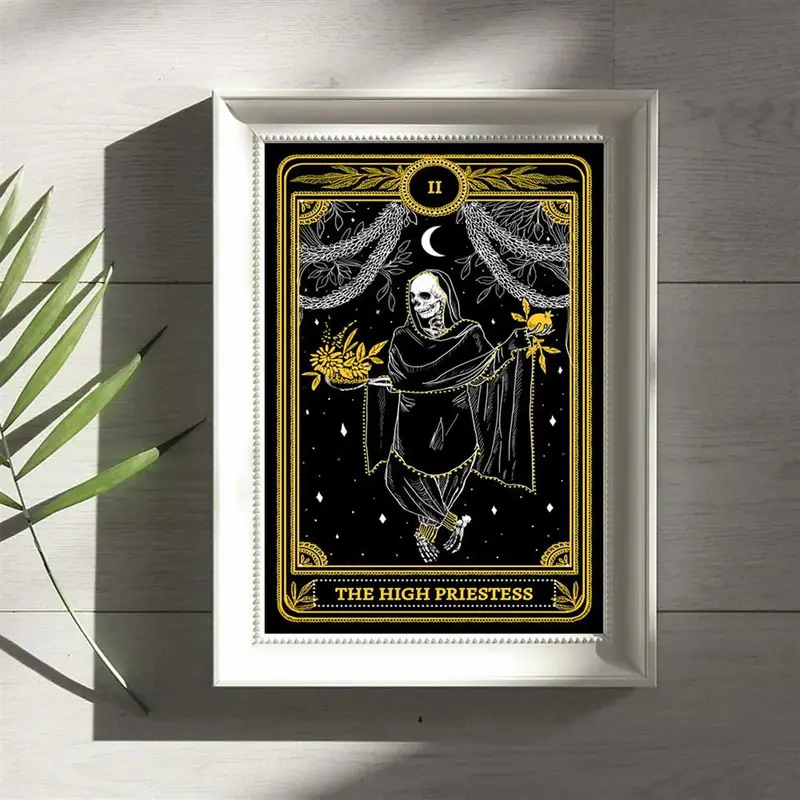This image depicts a flat lay of a framed tarot card and some greenery arranged on a wooden surface. The tarot card, encased in a sleek white frame, showcases an original interpretation of the High Priestess card. The design features a predominantly black background with intricate white lines and gold decorative elements. The High Priestess is depicted as a skeleton adorned in elaborate black robes with gold accents, holding a bouquet of flowers in one hand and a pomegranate in the other. The card is embellished with a crescent moon above the figure, diamond-like stars, and garlands of leaves and branches in the background. The Roman numeral II and the label "The High Priestess" are inscribed at the top and bottom of the card respectively. The framed image and a green palm frond are placed on a wooden floor with visible planks, adding a rustic touch to the setting.